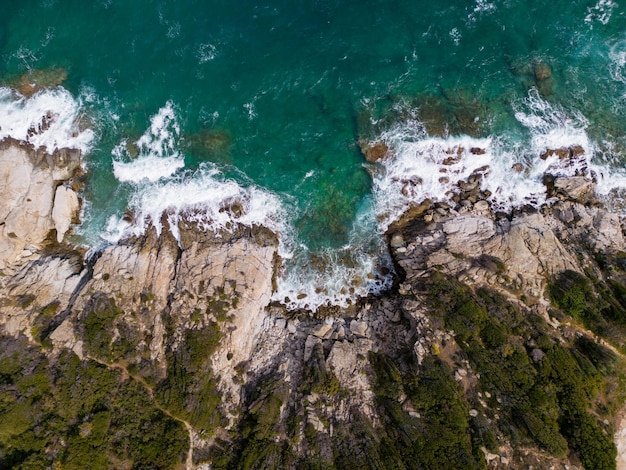The photograph appears to be an aerial shot taken from the top of a jagged, light brown cliff, although it may be upside down based on the orientation of the trees. At what appears to be the bottom of the image, or the upper part due to the potential flipped nature, lush green trees and possibly bushes line the edge of the cliff. The cliff face descends into tumultuous turquoise-green waters, where white waves crash against numerous rocks scattered along the shoreline. This dynamic scene, with its striking juxtaposition of rugged terrain and serene yet powerful waters, creates an impression of natural beauty and ancient geological formations. The vibrant colors and detailed textures of the cliffs, foliage, and waves suggest a clear, sunny day, enhancing the vividness of both the land and the sea.